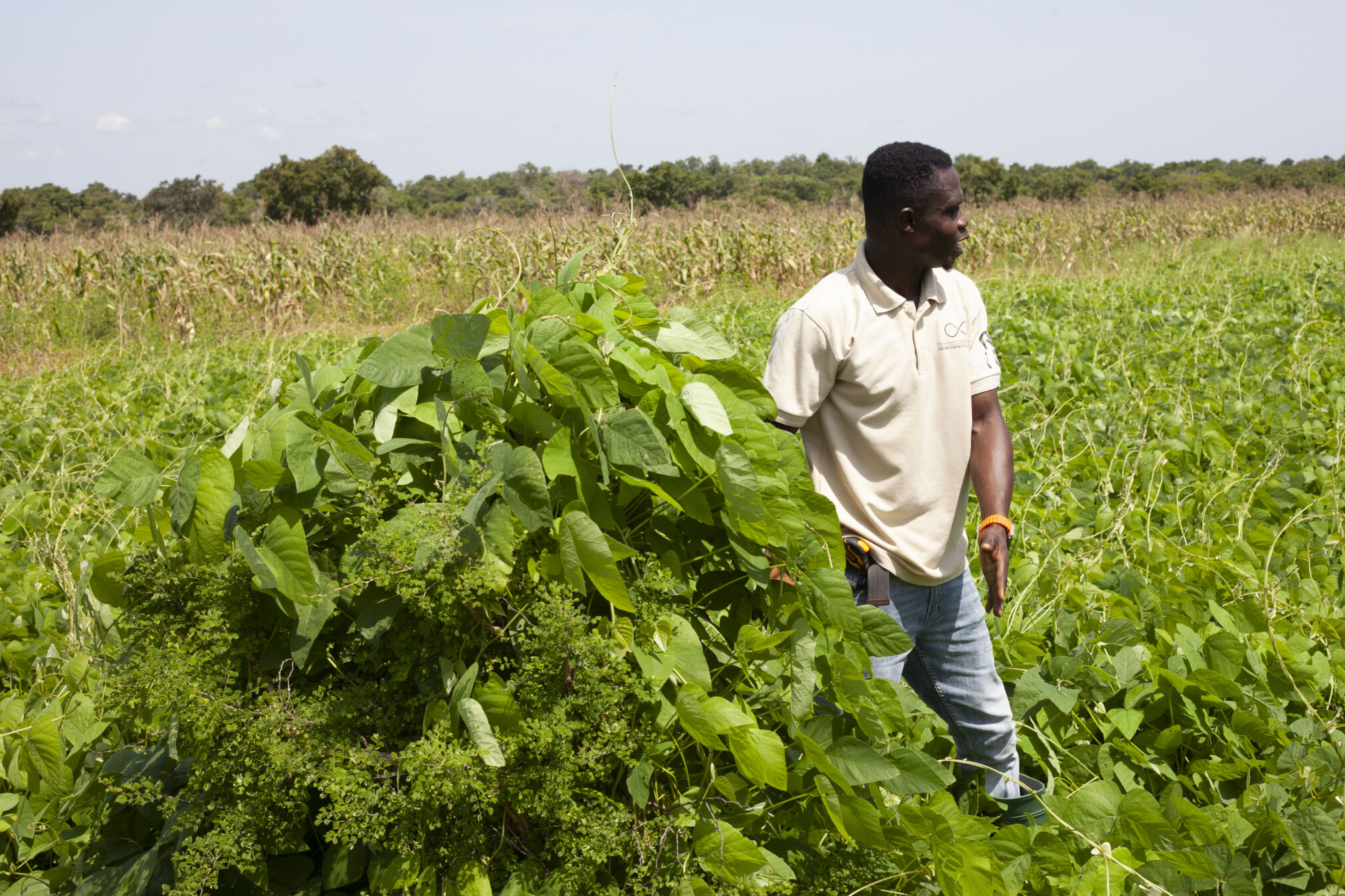In a sun-soaked, vibrant green field, an African-American man stands slightly right of center, surrounded by an abundance of lush, leafy plants. The dense foliage, featuring two or three different kinds of plants, rises to knee depth in some places and is piled up to his shoulder length nearby, suggesting he might have been working on removing weeds. He is dressed in a cream off-white polo shirt and light blue jeans, with a tape measure clipped to his hip and an orange band around his left wrist. His gaze is directed off to the right, presenting a thoughtful profile view. In the background, the greenery transitions to dried, crispy, brown leaves, and beyond that, rows of corn stalks stretch out towards the horizon where numerous trees stand under a bright, nearly cloudless sky. The brightness of the day accentuates the vivid colors of the scene, capturing the man's solitary presence amidst the thriving plant life.